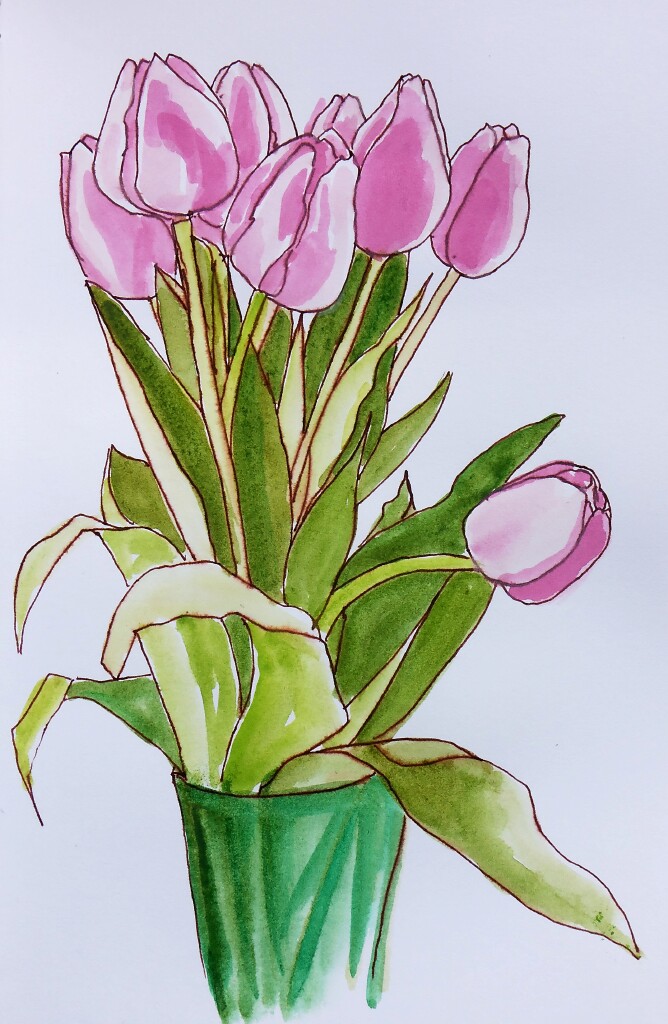A delicate watercolor painting features a blue glass vase positioned at the bottom of a white background. Rising vertically from the vase, five to six stems topped with vibrant purple tulip buds create an eye-catching profile view. The tulip arrangement includes seven buds, all pointing upwards, except for one distinct stem that bends to the right, showcasing a single tulip bud facing right. Interspersed among the stems are a mix of seven to eight vertical leaves in light and dark green hues. Notably, four to five leaves on the left side curl downward towards the lower left corner of the painting. This artwork captures the elegant simplicity of the tulips without any accompanying words, text, or signature.